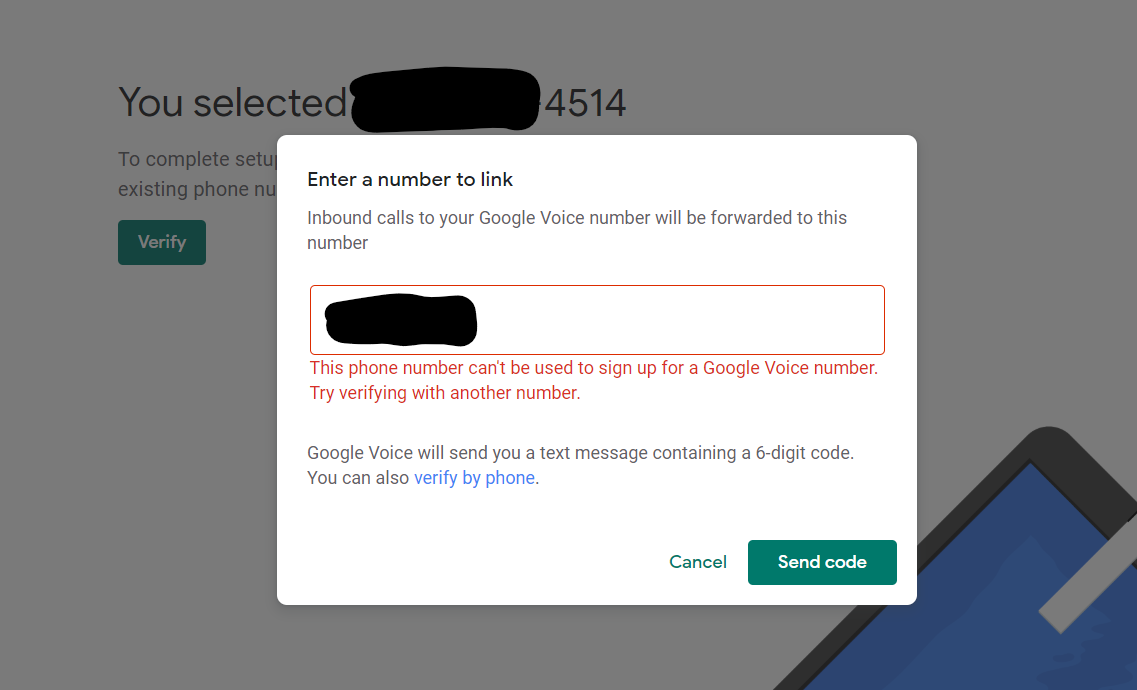The screenshot depicts a computer screen displaying a dimmed background with a central, prominent white dialog box. The white box commands attention with a header that reads, "Enter a number to link," and explains beneath it that inbound calls to a Google Voice number will be forwarded to the provided number. 

Inside the box, a notification bordered in red alerts the user: "This phone number can't be used to sign up for a Google Voice number. Try verifying with another number." The specific number has been obscured using a black Sharpie for privacy. 

Further instructions within the dialog state, "Google Voice will send you a text message containing a six-digit code," accompanied by a clickable, blue hyperlink that offers the alternative to "verify by phone."

At the bottom of the dialog, there are two actionable buttons: "Cancel", displayed in green text, and "Send code", rendered in green with white text overlay.

In the grayed-out background, there's additional text partially visible which reads, "You selected [blank] 4514," with another section obscured by a black marker for privacy purposes.